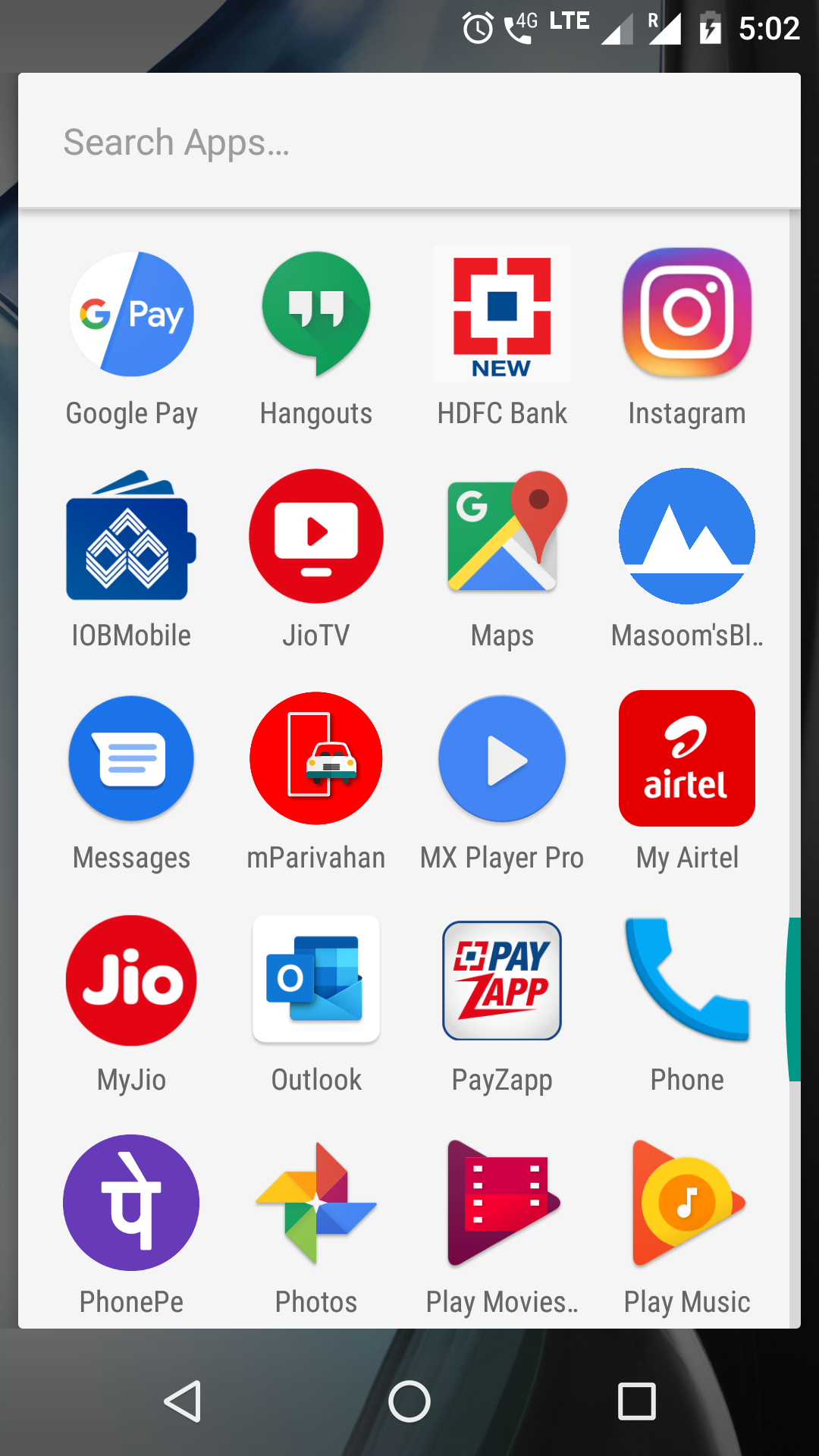This image is a detailed screenshot of a smartphone's home screen, featuring a dark grayish-black wallpaper. In the status bar at the top right, several icons are visible: an alarm clock emoji, a phone signal indicator showing 4G LTE, an almost fully charged battery icon, and the time "5:02." Below the status bar, there is a prominent search bar labeled "Search apps."

The main section of the screen is occupied by a grid layout of app icons arranged in five rows, with each row containing four icons:

**Top Row**:
1. Google Pay
2. Hangouts
3. HDFC Bank
4. Instagram

**Second Row**:
1. IOB Mobile
2. JIO TV
3. Google Maps
4. Me

**Third Row**:
1. Zoom
2. BL
3. Messages
4. M

**Fourth Row**:
1. Paravan
2. MX Player Pro
3. My Airtel
4. My JIO

**Fifth Row**:
1. Outlook
2. Hayzap
3. Phone
4. PE

At the very bottom of the screen, there is a dark background featuring three navigation buttons: a triangle pointing to the left (Back), a circle (Home), and a square (Recent Apps).